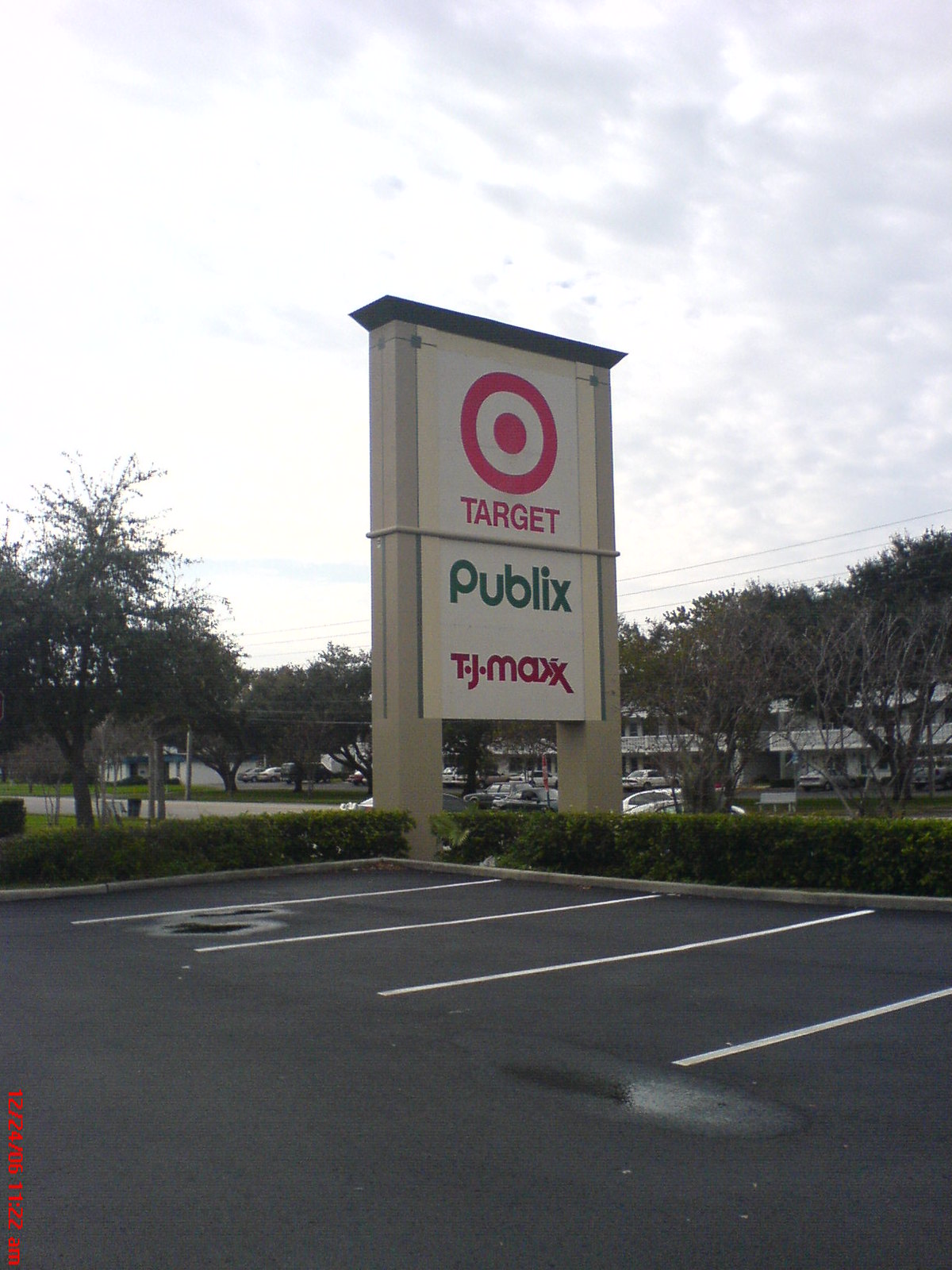This image captures a section of a spacious car park belonging to the companies Target, Publix, and TK Maxx, indicative of a substantial commercial complex. The foreground showcases several marked parking bays adjacent to a low, neatly-trimmed green hedge. Rising above the hedge is a distinctive noticeboard, reminiscent of the Arc de Triomphe's shape, featuring three divisions, each adorned with the logos of the respective companies. The background reveals a cluster of trees and various other buildings, reinforcing the sense of a larger commercial area. Numerous cars can be seen parked across the lot, extending to the point where the observer is standing. The Time Academy building is visible in a grey hue, adding to the architectural diversity of the scene. The sky overhead is partially cloudy, casting a diffused light over the entire parking area.